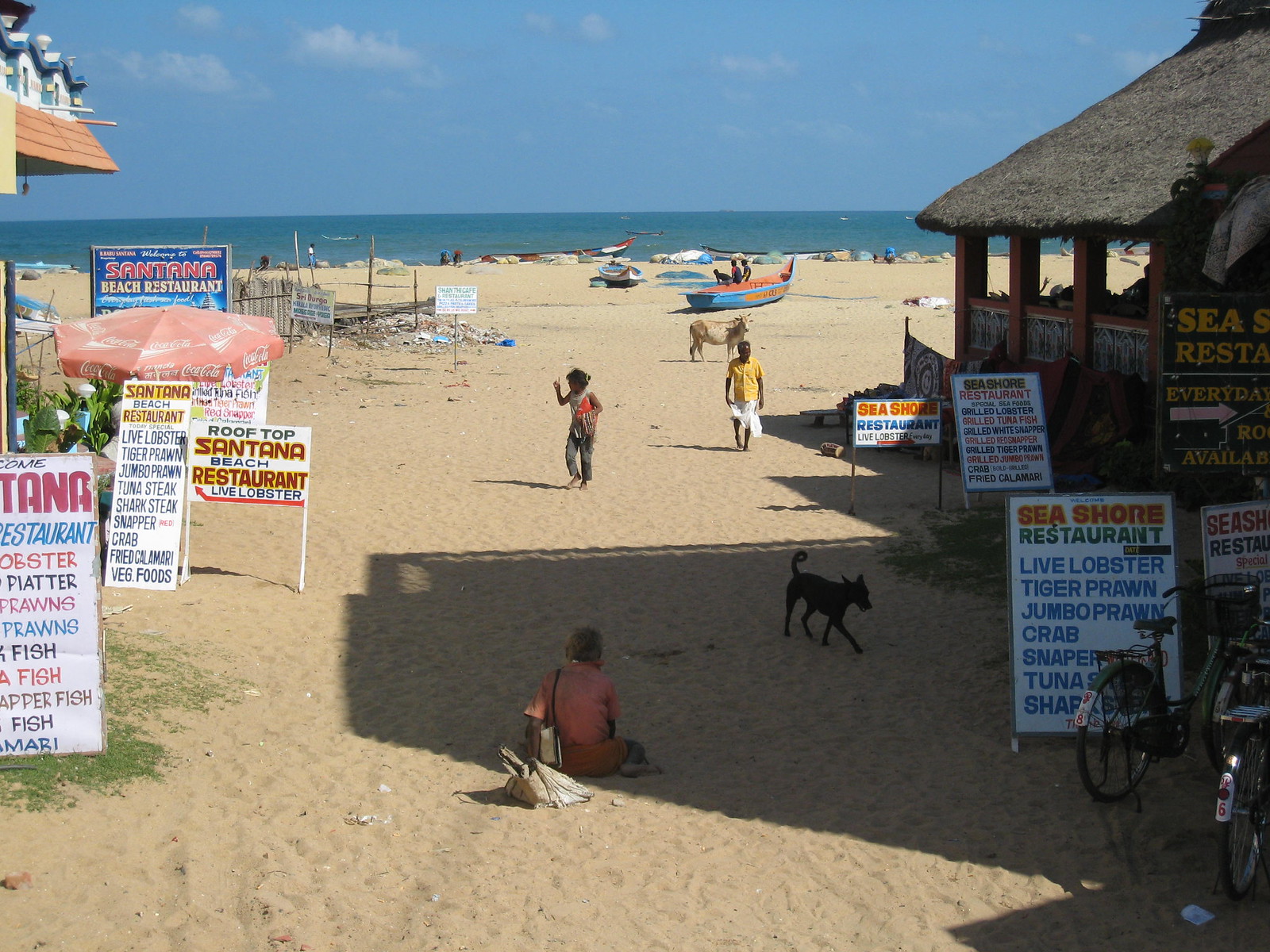In this image, a bustling beach scene unfolds under a vast sky. The sandy shore, which dominates most of the frame, appears somewhat cluttered with scattered trash, boats, and fishing nets. Scattered around the beach, a few people can be seen enjoying the seaside. More strikingly, a cow surprisingly roams the sands, adding an unusual element to the scene. To the left and right edges of the image, numerous signs advertise various seaside eateries and their offerings. Among them are "Seashore Restaurant" and "Santana Beach Restaurant," with menus boasting live lobsters, tiger prawns, jumbo prawns, crabs, snappers, and tunas. Nestled amidst these signs, a black dog is visible on the right, contributing to the overall commotion of this lively beachfront.